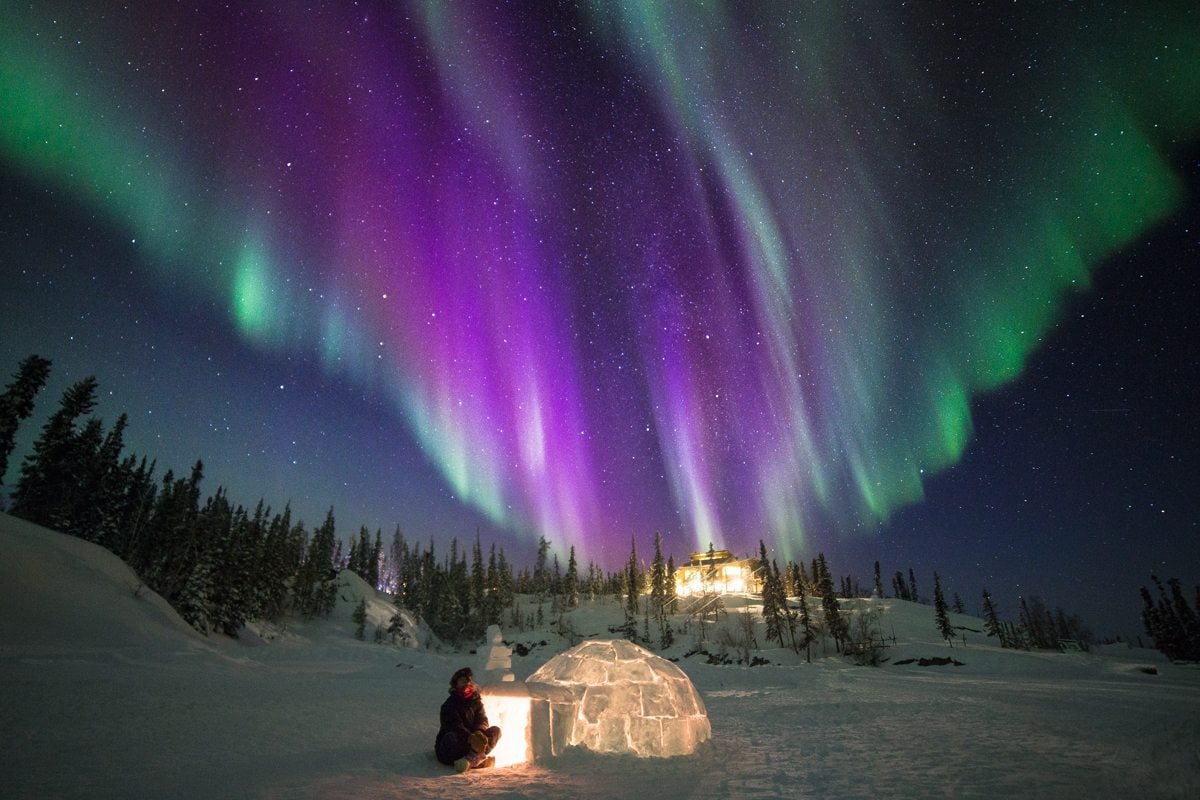This enchanting nighttime winter landscape is dominated by the mesmerizing northern lights, which fill the upper two-thirds of the image with spectacular streaks of bright green and purple, reminiscent of a science fiction scene. The ground below is coated in snow, scattered with evergreen trees creating a serene yet dramatic setting. Just in front of the illuminated snow-covered terrain stands an igloo, intensely lit from within, casting a warm glow on the surrounding snow. At the entrance of the igloo, there is a person, possibly engaged in some form of artistic activity, sitting amidst the captivating scene. In the background, a brightly lit structure, possibly a house, adds another element of intrigue to the landscape. The contrasting elements of artificial light from the structures and the natural brilliance of the northern lights create a picturesque and detailed winter wonderland.